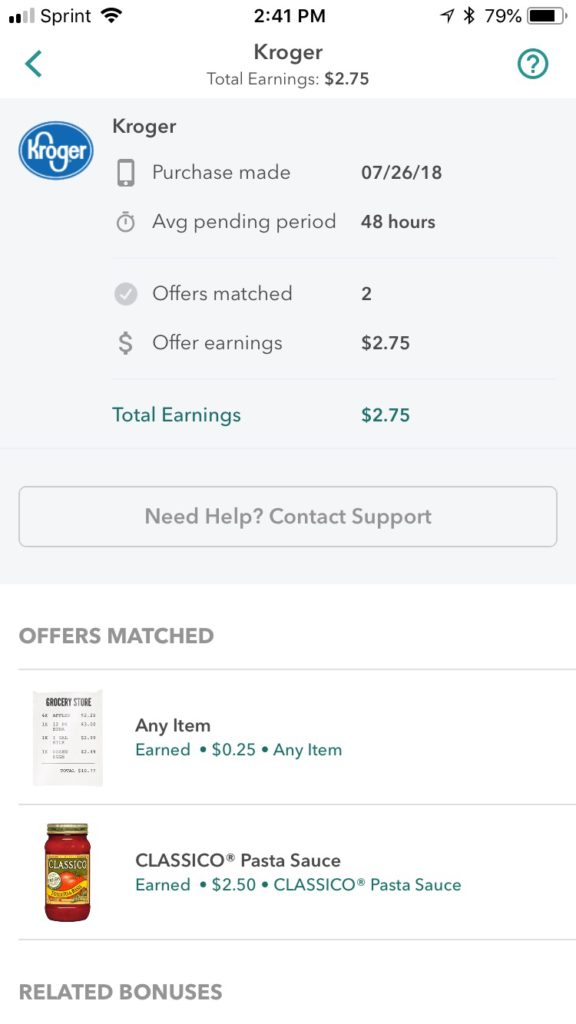A screenshot of a Kroger account page is displayed on a cell phone screen, which is connected to Sprint with two out of four signal bars and Wi-Fi. The time shows 2:41 PM, with the Bluetooth icon indicating an active connection, and the battery at 79% capacity. At the top, the Kroger logo is featured, followed by "Total Earnings: $2.75," suggesting participation in a rewards program. A green question mark encased in a green circle is present, likely offering additional page information. Below that, there's a yellow box featuring the Kroger logo in white script. The document details a purchase made on 07-26-18, noting the average pending period of 48 hours. The offers matched with offer earnings total $2.75, reflecting the customer's accumulated rewards.